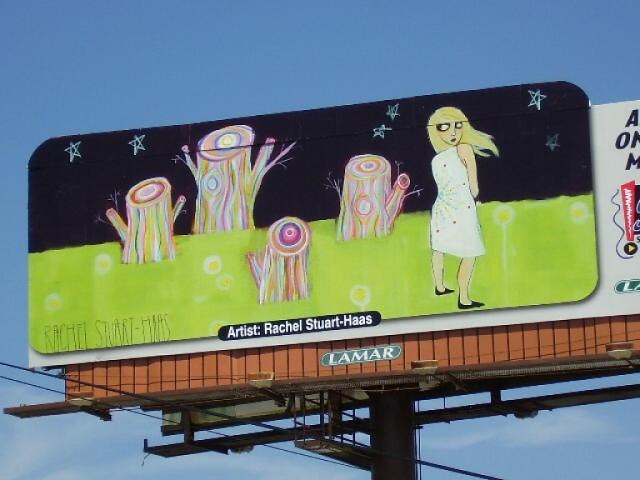A billboard stands against a vast blue sky dotted with fluffy white clouds, revealing its sturdy metal framing and the name "Lamar" at the bottom, indicating the likely owner. The focal point of the billboard is a captivating art piece by artist Rachel Stewart-Haas, as credited on the display. The artwork features a woman in a white dress and black shoes, standing in a grassy field. Her back is turned, but she glances over her shoulder, revealing her flowing blonde hair. The night sky behind her is illustrated with childlike five-pointed stars, evoking a sense of whimsy. Surrounding her are vibrant tree stumps, painted in an array of colors including pink, red, blue, and orange, adding to the enchanting and surreal atmosphere of the scene.